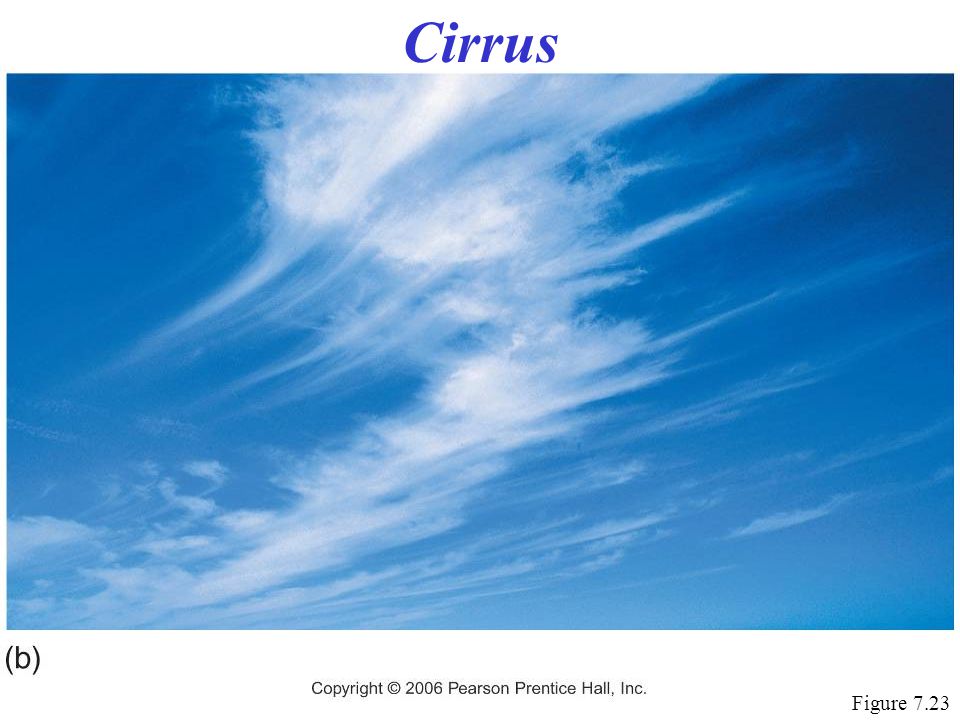In the image, we observe a thin, wispy Cirrus cloud extending from the top center down to the bottom center against a predominantly clear blue sky. The cloud is characterized by its delicate, linear edges, contrasting with the varying hues of purple, white, blue, gray, and black scattered across the sky. This image appears to be from an educational textbook, as indicated by the structured layout and specific annotations. At the top of the image, the word "Cirrus" is prominently displayed in bold blue text. Below the image, annotations include a lowercase 'b' in parentheses on the bottom left, the capitalized text "Figure 7.23" on the bottom right, and centrally placed text stating "Copyright © 2006 Pearson Prentice Hall, Inc."